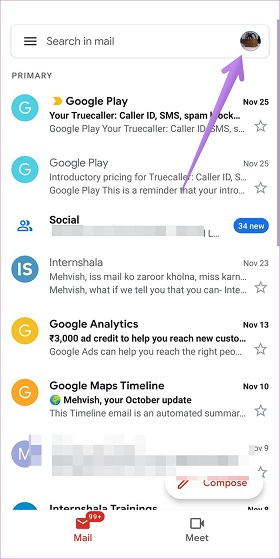This is a detailed screenshot of an email application displayed on a smartphone with a predominantly white background. At the top, there is a white search bar with a menu button located on the left and a circular profile picture on the right. The text within the search bar reads "Search in mail". A purple arrow points upward towards the profile picture, emanating from the bottom of the screen.

Below the search bar, five different emails are visible within the inbox. Each email entry features colored letters enclosed in circles on the left side, representing the sender's initials. Adjacent to these circles are the titles of the emails, followed by brief excerpts from the email contents. The dates of the emails are positioned on the right side of each entry.

The first email is from Google Play, titled "Your True Caller ID, SMS, Spam Block". The snippet from this email reads "Google Play, your true caller ID, SMS". The date of this email is specified as November 25, and there is a star icon next to the date, presumably for marking the email as important or favorite.